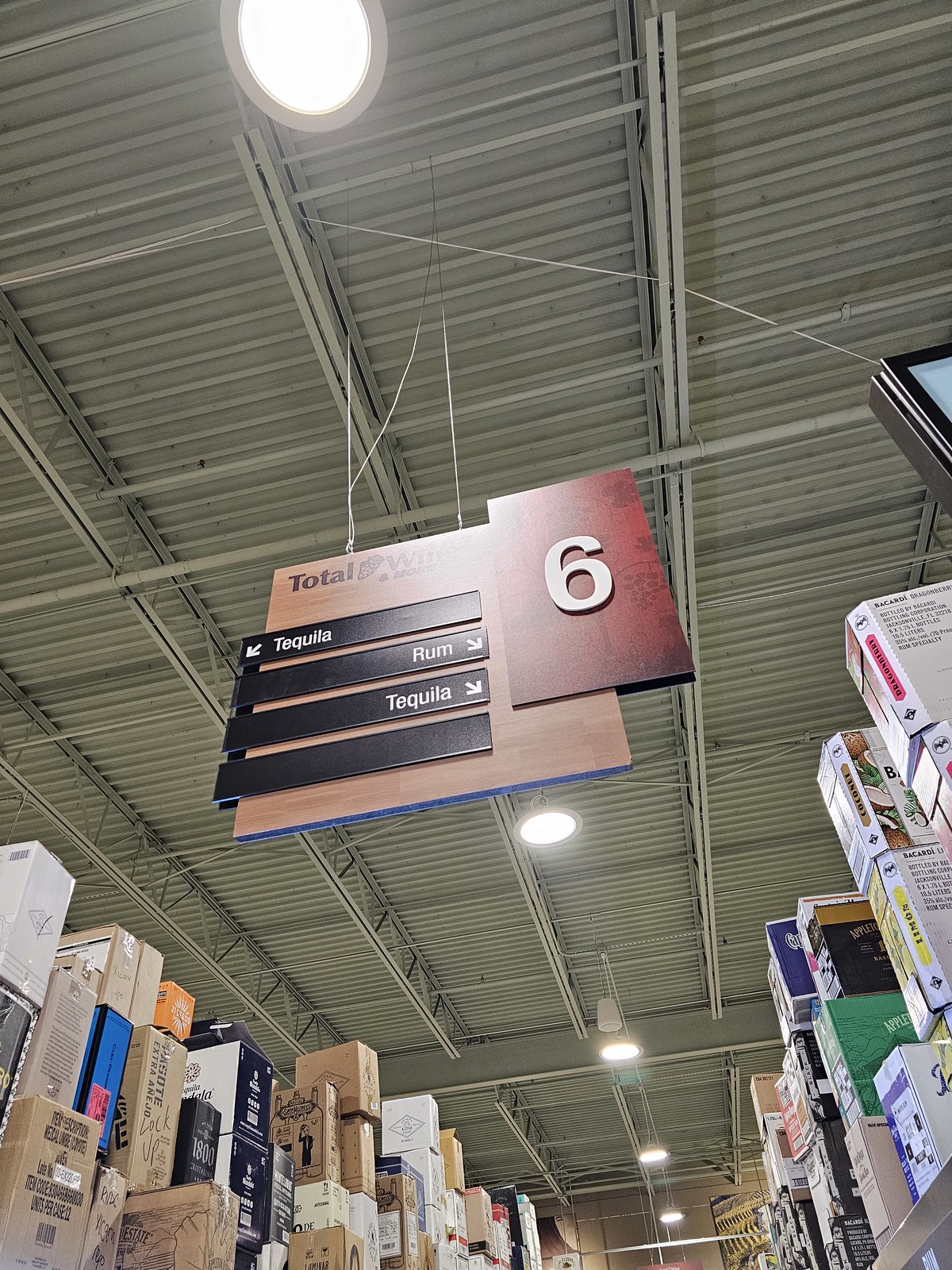The photograph depicts an aisle sign in a warehouse-style store with a metal roof and exposed rafters. Large LED lights hang from the ceiling, illuminating stacks of boxes in various colors and sizes. On the left, the boxes are haphazardly piled, while on the right, they are organized on metal shelves. The sign at the center is a tan wood square with a smaller reddish rectangle on the top right, displaying the number six in white. Four black bars run across the sign horizontally. The top bar reads "tequila" with an arrow pointing down and to the left. The second bar reads "rum" with an arrow pointing down and to the right. The third bar also reads "tequila," with an arrow pointing down and to the right, while the fourth bar is blank. This signage indicates the aisle's contents, suggesting it holds different types of alcohol. The variety of boxes below further adds to the store's eclectic vibe.